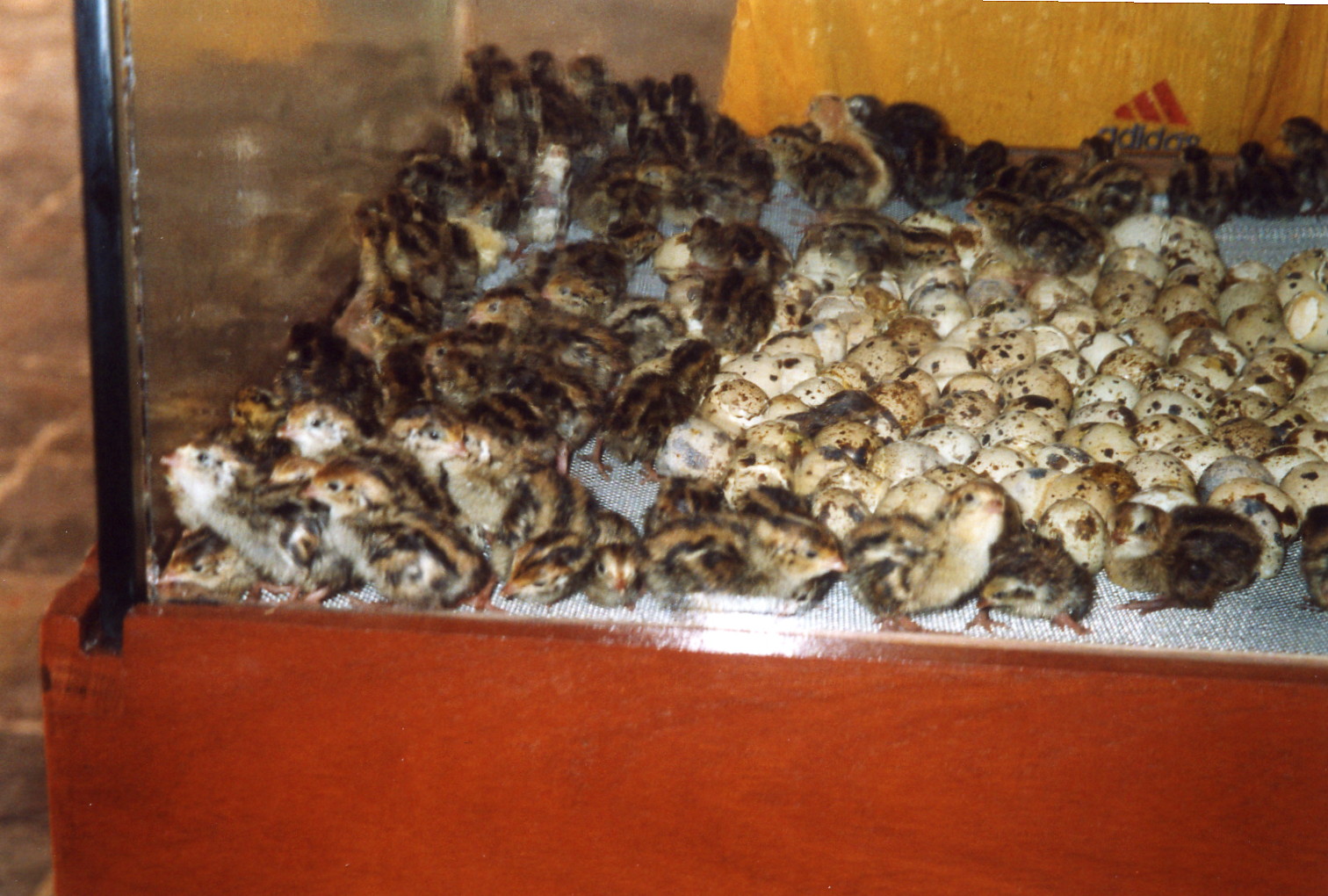The photograph captures a somewhat unsettling scene of a glass enclosure densely populated with numerous small chicks and a sizable collection of eggs. The chicks, characterized by their fluffy bodies with various shades—brown, white, black, and striped black bodies with brown fur—are huddled near the corners of the tank, suggesting their desire to escape the cramped space. The eggs, many of which have already hatched, are scattered mainly on the right side of the image. These eggs are notably different from typical store-bought eggs, with dirty, beige, brown, and speckled shells, some appearing soiled. The enclosure has a wooden panel at the bottom and a metal-grated floor, providing an industrial feel. Additionally, a white cloth or bag, potentially a t-shirt with an Adidas logo, is visible in the background at the top right of the image. The thick glass panel on the left side of the frame and the crowded condition of the chicks add to the overall bleak impression of the scene.